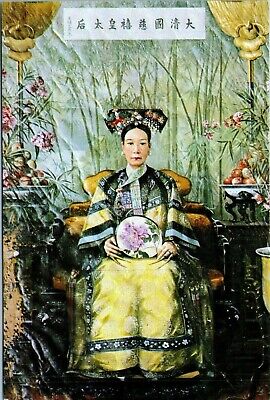This image depicts an intricate painting of a Japanese woman, possibly a geisha or noble figure, seated gracefully against a backdrop of lush bamboo and vibrant pink flowers. She is adorned in a luxurious yellow kimono, embellished with black stripes and gold accents, which flows elegantly around her. Her attire includes a headdress, with her black hair pulled back, and she wears traditional geisha makeup. Remarkably long, sharp nails, possibly with finger covers, add to her distinguished appearance. In her hands, she delicately holds a circular embroidery frame showcasing a purple flower. Surrounding her are elaborately carved tables adorned with bowls of fruit, enhancing the opulent setting. Above her, a white banner displays black Chinese calligraphy, adding a cultural and historical element to the scene. The overall setting and details reflect a harmonious blend of natural beauty and regal elegance.